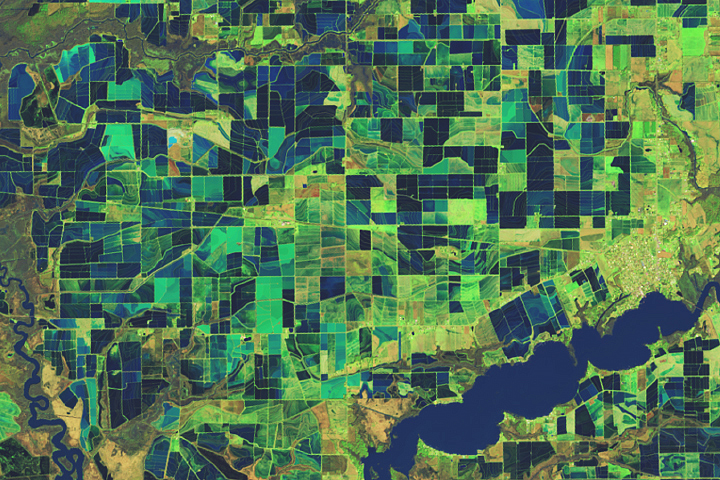This image is an overhead, aerial view resembling satellite imagery, displaying a detailed map of a region. Dominating the bottom right of the image is a deep midnight blue waterway, surrounded by numerous rectangular and square plots in various shades of green and blue, closely resembling farmland sections. These plots are meticulously sectioned off and scattered across the landscape, creating a mosaic pattern. The different shades of green suggest grassy areas, more concentrated in the mid-right section of the image. Towards the left and top, the plots shift to darker navy and midnight blue hues. The lake's irregular shoreline is dotted with islands and coves, enhancing the intricate details of the mapped region. Though the image lacks a legend, the contrasting colors and sectioned plots effectively highlight the diverse landscape features and land use.